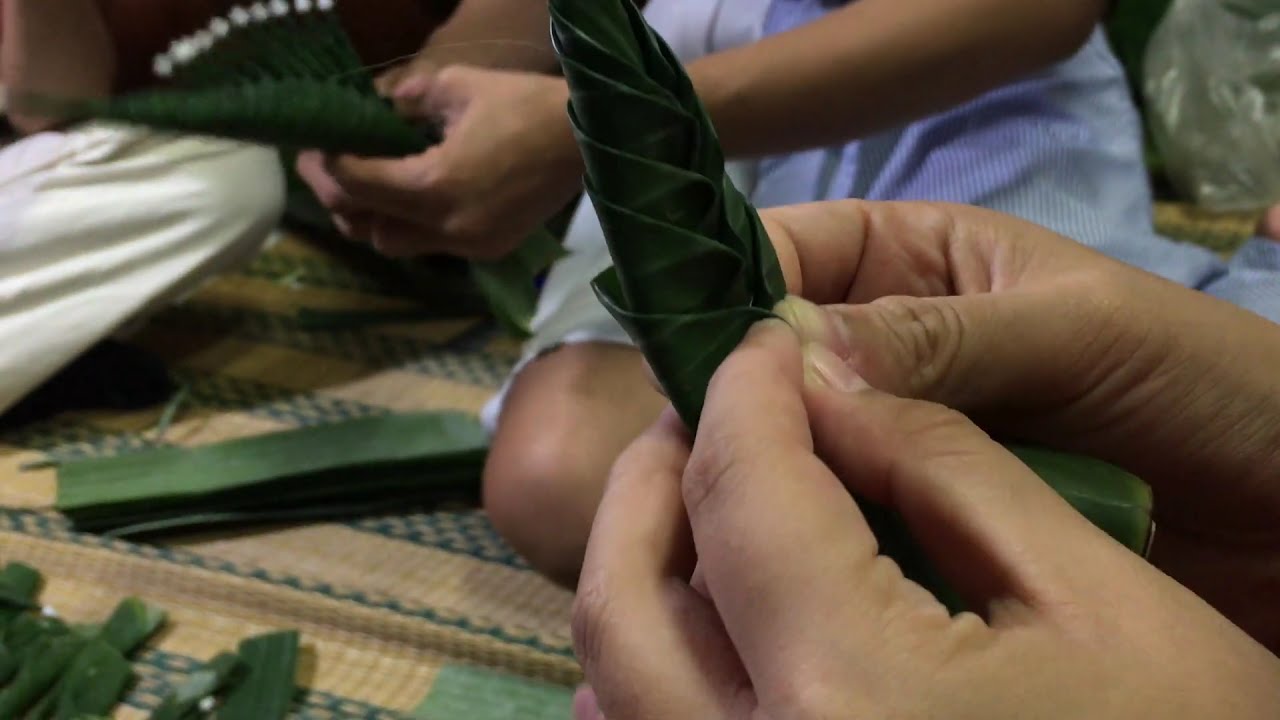In the image, we see three individuals seated on a tan and green checkered carpet indoors, engaged in a meticulous arts and crafts activity involving green leaves. They are folding these leaves, which are either plant leaves or green rectangular paper, into some elaborate shapes. Piles of these folded parts can be seen in the lower left corner, and fresh leaves or paper sheets are stacked above them, ready for use.

The participants' hands are light brown in color and actively shaping the leaf structures. One female participant is wearing a purple dress or skirt, and another individual is sporting white pants. Additionally, there's a person with visible arms dressed in blue attire with slight white stripes, although their top half is obscured.

In the upper right, there is a bag behind one of the participants. The hands closest to the camera appear adult-sized, while another set of hands seems smaller due to perspective. The setting clearly indicates a collaborative and creative environment, with the participants deeply engrossed in their leaf-folding project.